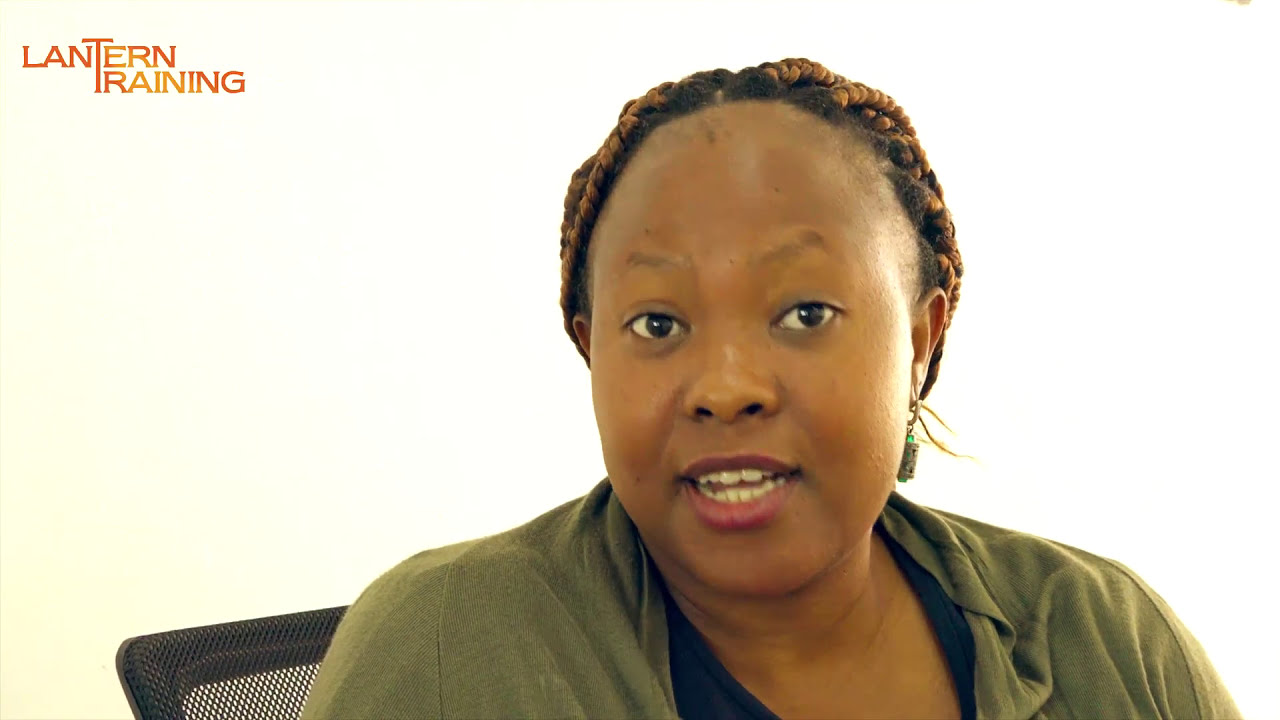In the image, we see an African-American woman sitting in a black mesh-backed chair, facing the camera, and appearing to speak. She has cornrows, which are tied back, with her hair showing a hint of an orangish tone. Her high forehead is complemented by very thin or almost non-existent eyebrows. She wears purple lipstick, and her mouth is slightly open, revealing both her teeth and a bit of her tongue, indicating she is mid-sentence. She's adorned in a green long-sleeved sweatshirt over a purple blouse, with a dangling earring decorated with green stones. The background is a very pale peach or white-pinkish color, and in the top left corner of the image, there is a logo for Lantern Training with the words "Lantern Training" where the "T" is shared between the words. Overall, the woman appears to be engaged in speaking, likely in a training or instructional setting.